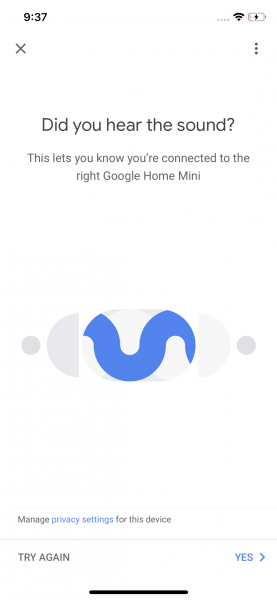The screenshot, taken from a smartphone at 9:37 AM while plugged into a charger (indicated by the battery icon with a lightning bolt), showcases a page within the Google Home app. The app is displaying a message: "Did you hear the sound? This lets you know you're connected to the right Google Home Mini." This screen helps users confirm the connection to their Google Home Mini device. It features a dynamic blue waveform design in the center, which likely animates when sound is played. Below the message, there's an option to "Manage privacy settings for this device," along with a "Try again" button. In the bottom corners, there are interactive options: a clickable "Yes" button in blue on the right and possibly another button on the left. The app is designed to assist users in linking their Google Home Mini to their home network, enabling them to utilize voice commands for accessing information like weather, time, temperature, and general queries, akin to a search engine.